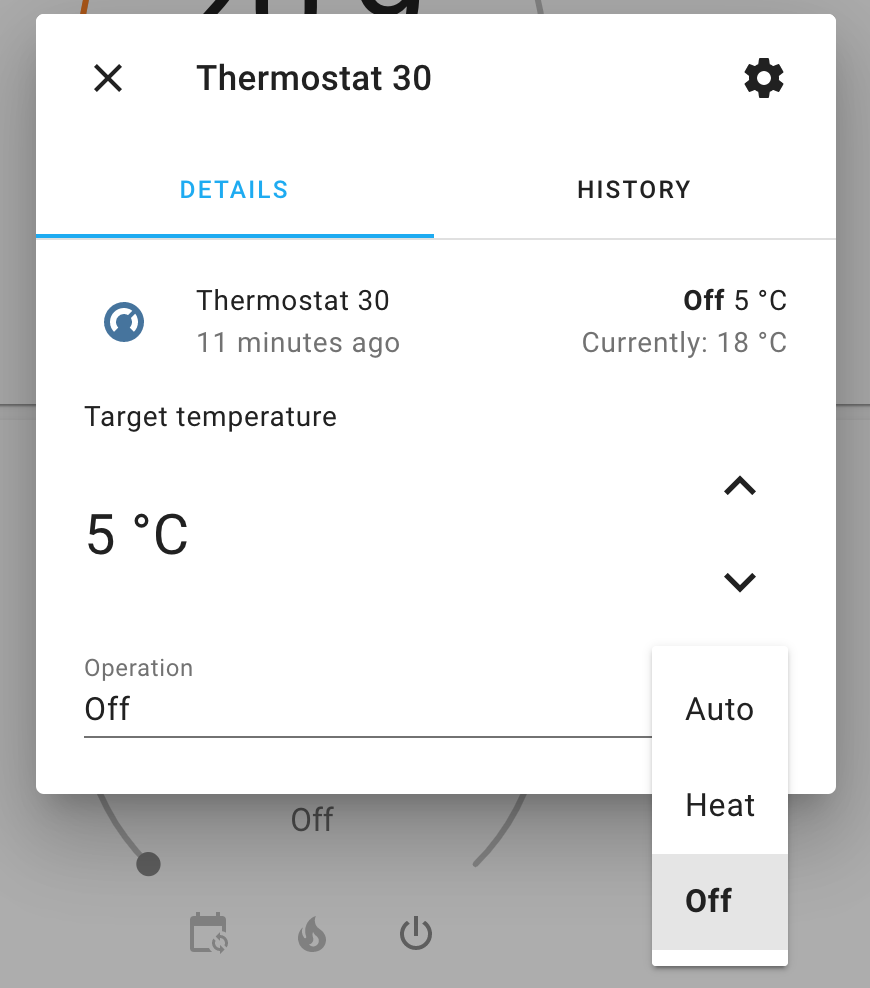The image depicts a digital interface, likely from a thermostat control application or website. The aspect ratio suggests the image is approximately 30% taller than it is wide. The background appears to be gray, indicating the presence of a secondary window behind the primary display, which is semi-transparently visible.

The secondary, background window has limited visibility but appears to show a thermostat interface. At the bottom, there are three icons: a document page, a flame symbolizing heat, and a power icon. The mode is set to "Off."

The foreground window occupies the top 75% of the image with a white background. In the top left corner, there is an "X" icon, indicating the option to close the window. Adjacent to it is the label "Thermostat 30" which identifies the device or interface in focus. The top right corner features a settings gear icon.

Approximately 25% down from the top, two menu options are aligned horizontally: "Details," highlighted in blue with an underline, and "History," in black with a gray underline, indicating that the current view is the "Details" page. Below this navigation, it reads "Thermostat 30, 11 minutes ago."

To the left, a dark blue icon with a cancel symbol indicates a restriction or prohibition, and to its right, the status "Off" is displayed with "5°C." Further down, in gray text, it states the current temperature is "18°C."

At the bottom, the left side of the interface provides information on the target temperature, showing "5°C."

Overall, the image presents a detailed view of a thermostat control interface, emphasizing both the current settings and historical context.